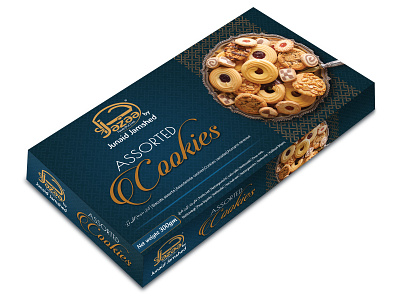The image features a 300-gram box of Jazaa by Junaid Jamshed Assorted Cookies. The rectangular box, turned at an angle, is a striking deep blue, almost dark teal color, adorned with elegant gold and white lettering. On the left side of the box, the brand name 'JAZAA' is prominently displayed in gold letters, while 'Assorted Cookies' appears in white. To the right, a vivid photograph showcases a variety of cookies, arranged in a bowl. These cookies come in various shapes and sizes, including rounds, squares, and spirals, with some featuring intricate swirls and checker patterns. Notably, several cookies have fruit or jelly fillings in the center, and some round ones bear unique imprints, possibly of a tree or other designs. Additional images and the same descriptive text are found on the narrow sides of the box, making the packaging visually appealing from multiple angles.